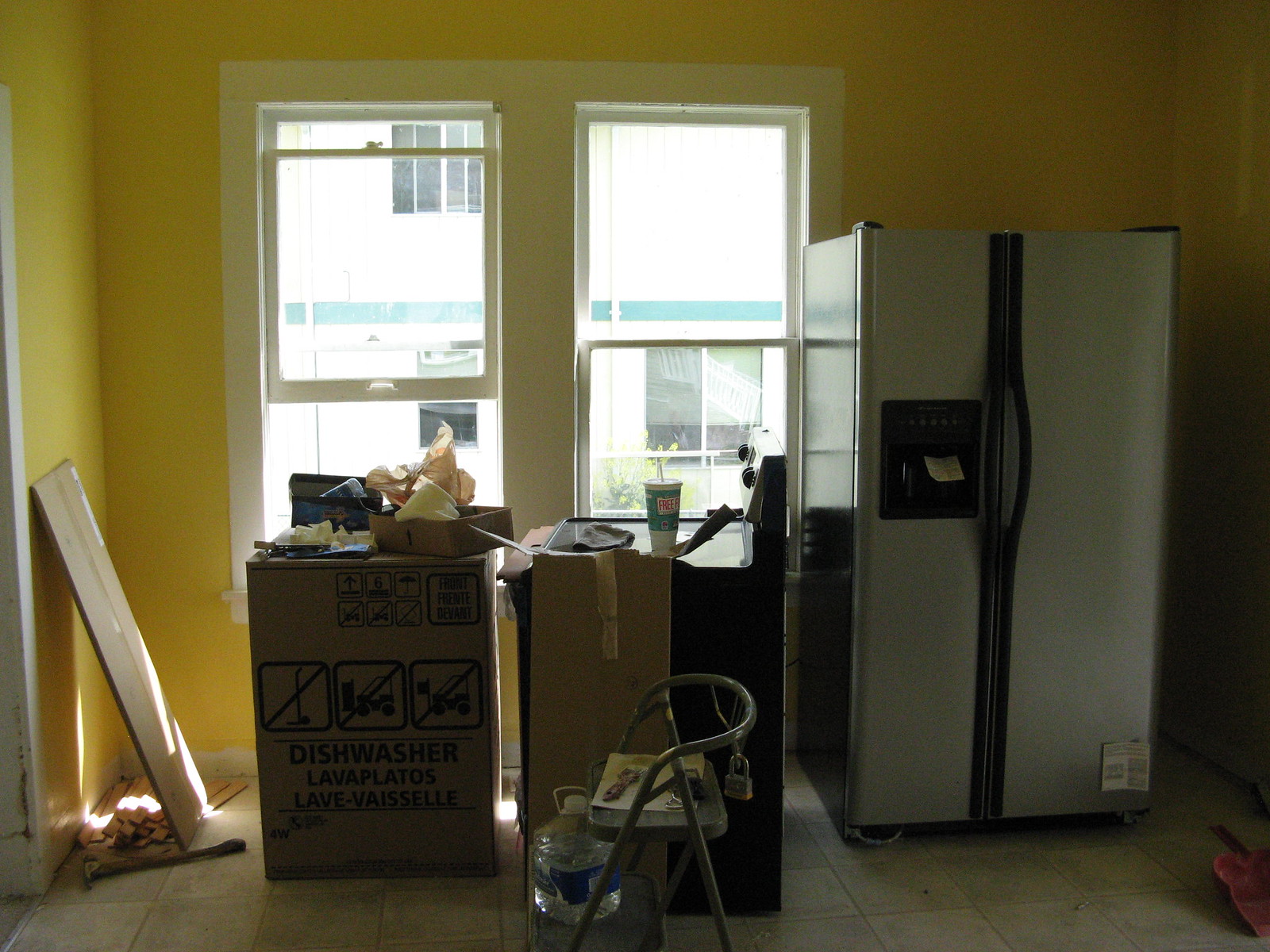The photograph captures the kitchen of what seems to be a recently occupied apartment. Positioned on an upper floor, the view through the open left window reveals another apartment building, indicating the elevated location. The kitchen is in the midst of being set up, with a prominent dishwasher box and an unpacked oven/stove unit taking center stage. A painter's stepstool, holding an almost empty 2-gallon jug of water, stands nearby. The kitchen also features a new two-door refrigerator in a sleek grey and black finish. 

To the left, a 1-inch thick wooden plank leans against the freshly painted yellow wall, accompanied by a hammer lying on the floor. Paint stirring sticks are partially visible behind the wooden board. Despite the fresh yellow paint dominating most of the wall, the area around the windows remains unpainted, exposing the bare drywall. The absence of window blinds further emphasizes the in-progress state of the kitchen renovation. On the right side of the image, a dustpan partially enters the frame, with the lighting on this side appearing darker compared to the left. The overall scene portrays the dynamic and busy nature of moving into and setting up a new apartment.